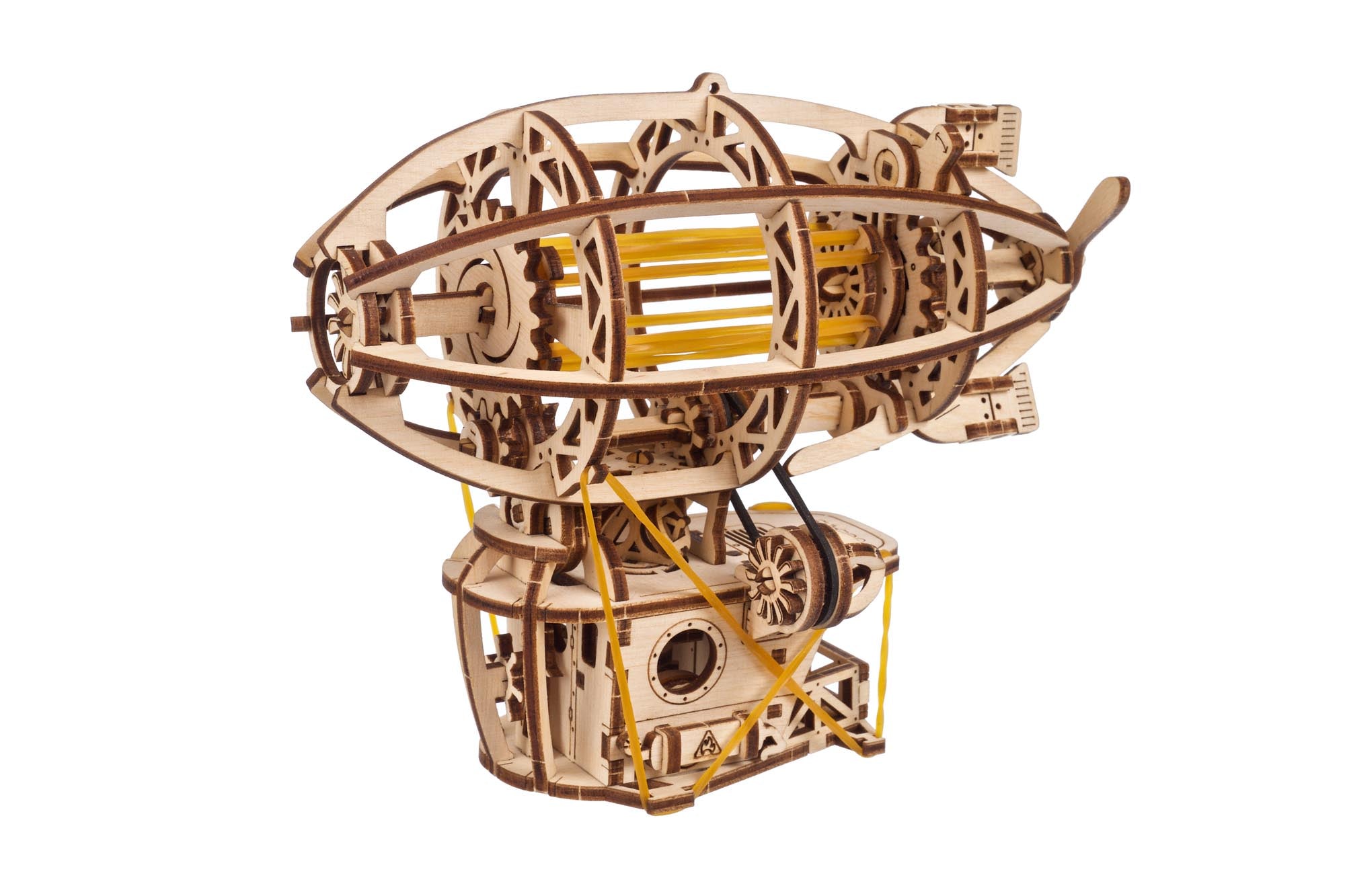The image shows an intricately designed, gold-colored object with a mechanical base. The base features a circular gear, visible through a small transparent section. Resting atop the base is a framework reminiscent of a blimp's silhouette, constructed from gold wire and adorned with additional gear elements. The overall structure combines an industrial and steampunk aesthetic, with the metallic tones and visible mechanical parts creating a sense of meticulous craftsmanship.